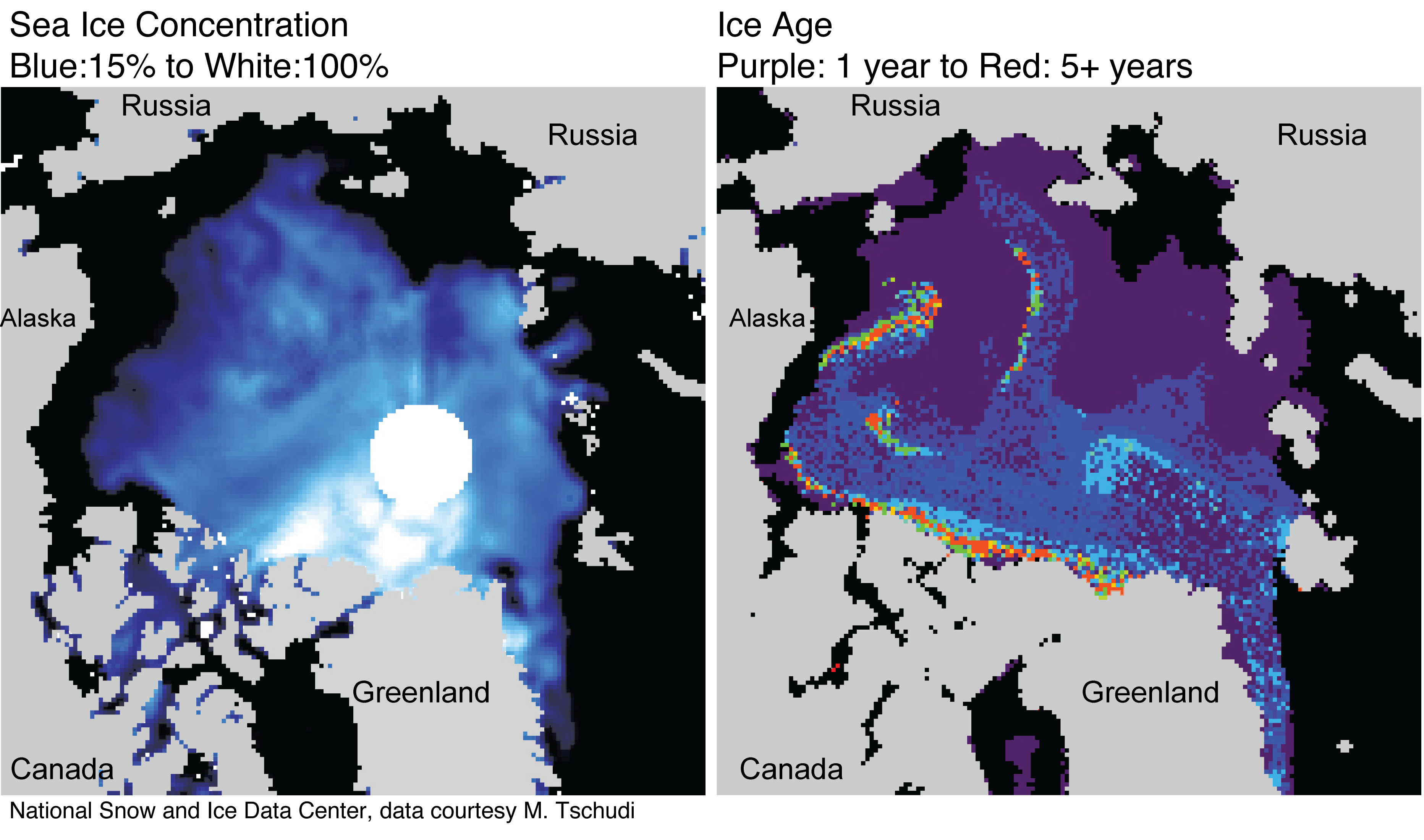This digital image consists of two side-by-side overhead satellite view maps illustrating the Arctic region, specifically between Alaska, Russia, Greenland, and Canada. The left map, titled "Sea Ice Concentration," uses a gradient from blue (15%) to white (100%) to show varying concentrations of sea ice. The right map, labeled "Ice Age," utilizes a color scale from purple (1 year) to red (5+ years) to depict the age of the ice. Both maps feature detailed overlays: the left map with shades of blue and white, while the right map showcases a mix of purple, dark blue, red, and green. The images are pixelated where the ice is present, reflecting accurate data from the National Snow and Ice Data Center. These highly detailed scientific illustrations are likely used for educational purposes, such as in textbooks or informational reports, to present data on the state of sea ice in the Arctic region.